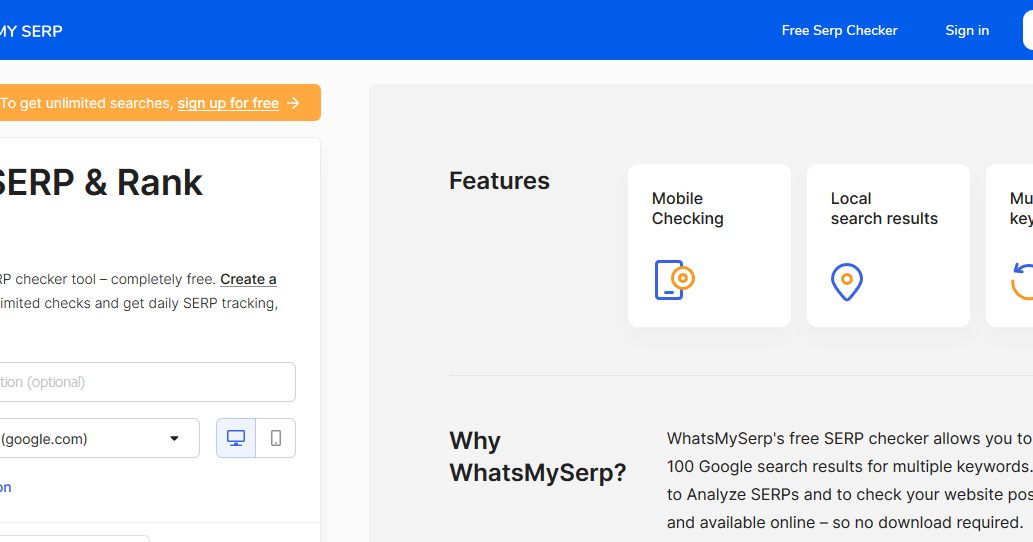A detailed caption for the described image could be:

---

The webpage from the website MySERP features a prominent blue border at the top, with the site name "MySERP" displayed in white text. To the right, the page displays options for "Free SERP Checker" and "Sign In." Beneath this header, there are several tabs starting with "Features," followed by "Mobile Checking" and "Local Search Results," though some text is cut off and not visible.

Below the tabs, partially obscured text reads, "Why? Why? What's MySERP? What's MySERP's Free SERP Checker Allows You To..." This is followed by more text cut off mid-sentence that seems to explain, "100 Google Search Results For Multiple Keywords To Analyze SERPs And To Check Your Website Posts And Available Online So No Download Required."

On the left side, an orange box with white text reads "To Get Unlimited Searches, Sign Up For Free," accompanied by a right-facing arrow. Below this, another segment with black text contains the headings "SERP" and "Rank" with partial text "SERP Checker Tool - Completely Free. Create a..." and further cut-off text mentioning "Limited Checks And Get Daily SERP Tracking."

The page also includes an "Optional" box, from what is readable, followed by another box with a drop-down arrow that states "Google.com" in parentheses. Finally, near the bottom, there are icons for a computer monitor and a smartphone, with the computer monitor icon highlighted.

---

This version maintains detail while organizing and clarifying the information for better readability.